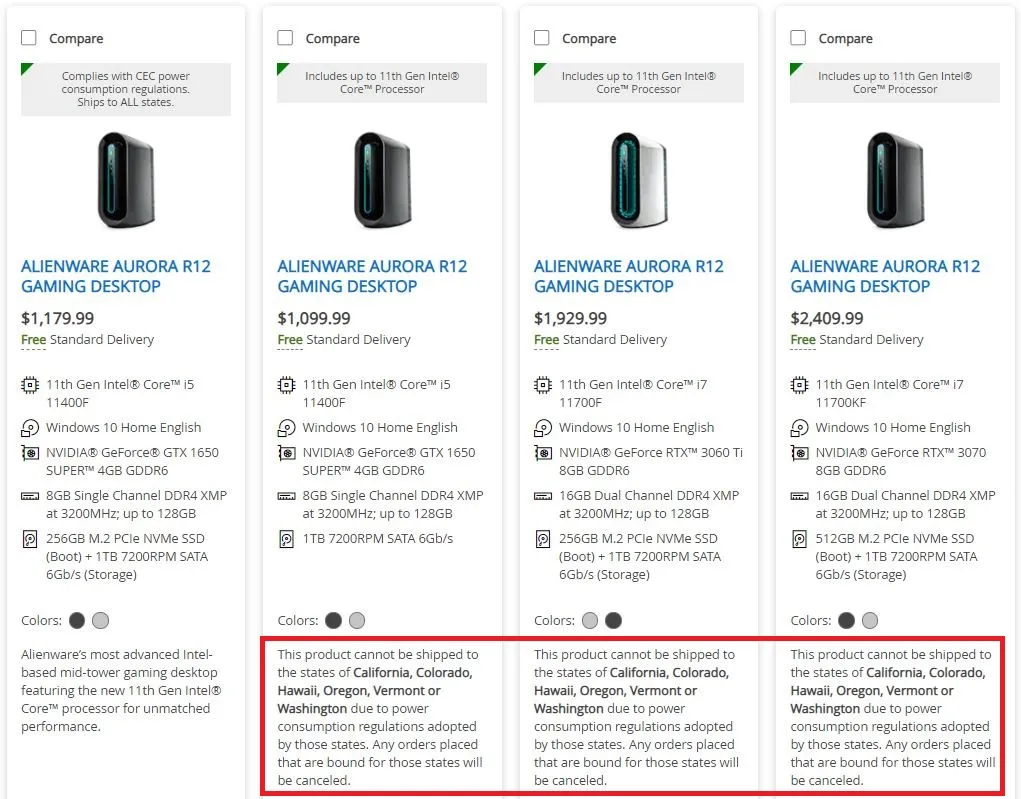The image depicts a comparison of four gaming desktop computers, organized in long, narrow strips. At the top, a header reads "Compare." Below each strip, there's a detailed description and price for each computer, ranging from $1,099.99 to $2,409.99. 

The leftmost strip highlights the Alienware Aurora R12, featuring an advanced Intel-based mid-tower gaming desktop with the new 11th generation Intel Core processor, promising unmatched performance. 

The next three strips, moving right, have a prominent red box added via photo editing at the bottom. This red box contains a notice stating: "This product cannot be shipped to the states of California, Colorado, Hawaii, Oregon, Vermont, or Washington due to power consumption regulations adopted by those states. Any order placed that are bound for those states will be canceled."

Notably, this shipping restriction applies to both the least and most expensive models shown in the comparison.